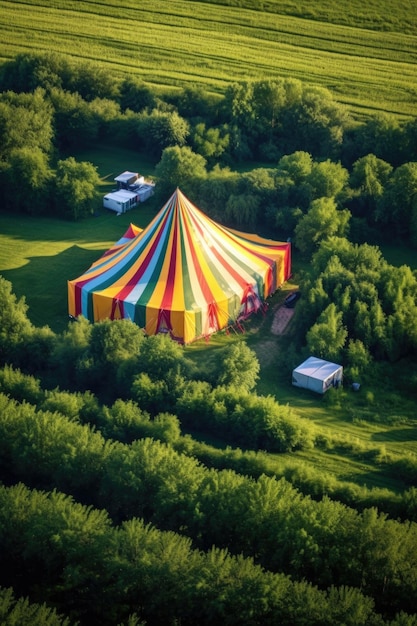A detailed aerial view captures a striking, multi-colored circus tent in the middle of a lush, green landscape. The tent, taller than it is wide, features bold stripes of red, yellow, green, blue, orange, and white, converging into the center and extending outward. The vivid colors make the tent stand out prominently against the green surroundings. Encircling this main tent are a few smaller, square-shaped structures and habitats, one of which is a light blue, and others are white support tents. These structures are scattered within a well-maintained, perfectly green mowed lawn that is surrounded by dense rows of trees and bushes, adding to the sense of isolation in this otherwise natural setting. The scene appears to be set in the middle of nowhere, with no signs of a town or human activity nearby, focusing entirely on the impressive, colorful circus tent amidst the rich greenery.